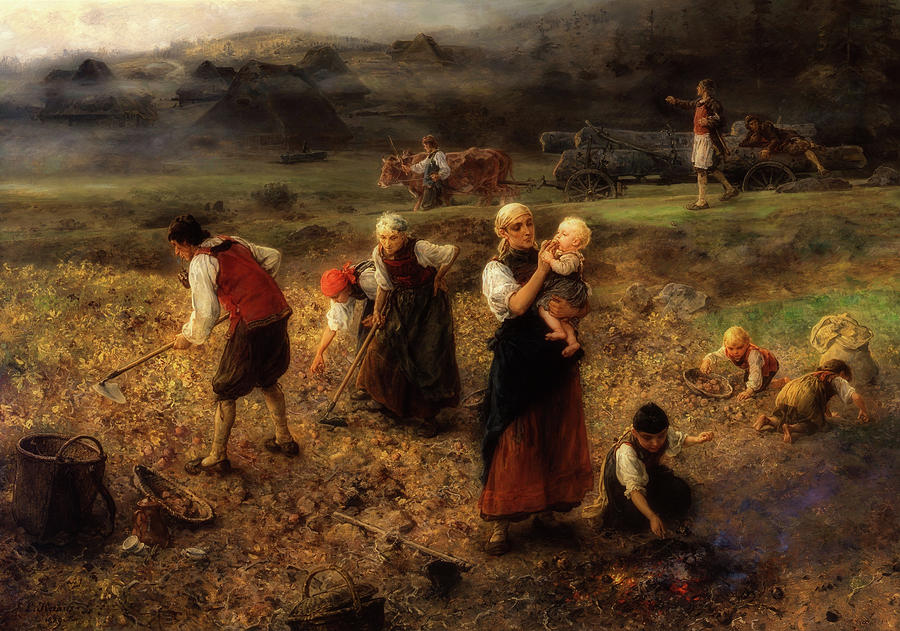The oil painting depicts an intricate scene of agricultural labor, where men, women, and children are actively working on a field. The foreground prominently features a small child who appears to be tending to a fire with some coals, while a nearby woman is delicately holding and feeding an infant. Three children are engaged in meticulously picking items—perhaps stones or potatoes—and placing them into a basket. Centered in the composition, men and women wield farming instruments, intensely focused on cultivating the land. To the far left, a man uses a large pointed digger to turn the soil, accompanied by a woman engaged in a similar task. Behind this bustling group, a bullock cart laden with lumber is managed by two people, with an additional person reclining on top of the load. The backdrop offers a glimpse of several large, triangular houses that are predominantly roofed, nestled amidst patches of green grass and yellow fields, enriching the pastoral landscape.